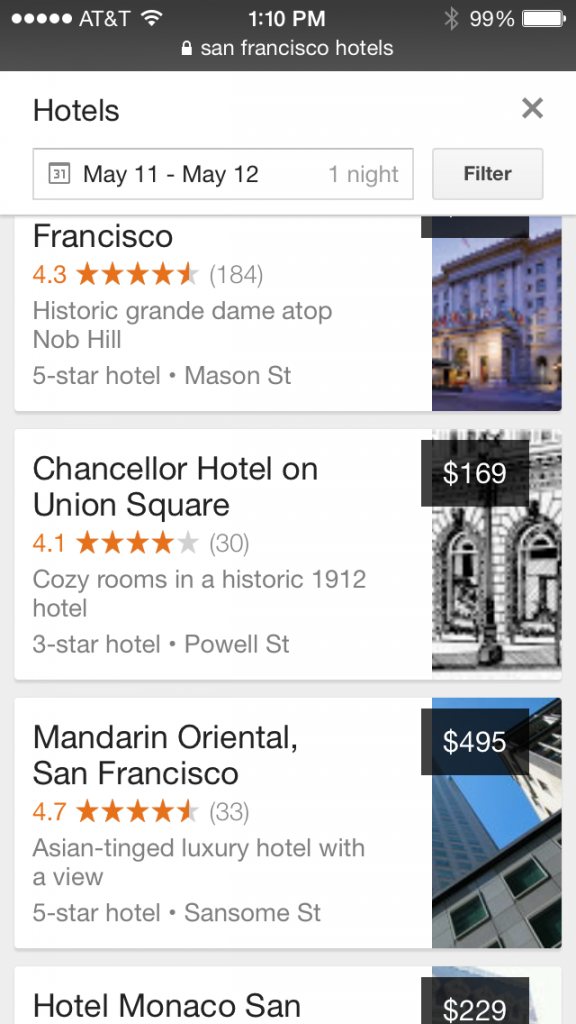The image captures a screenshot of a smartphone search for hotels in San Francisco. At the top of the screen, the status bar displays icons for AT&T, a full Wi-Fi signal, the time (1:10 PM), and a battery level of 99%. The YouTube app is not active. 

The search query entered is "Locked San Francisco Hotels," appearing above results listed against a white background. The search is filtered for the dates May 11th to May 12th, a one-night stay. 

The first hotel listed is the "Historic Grand Dame" atop Nob Hill, a 5-star hotel located on Mason Street. It has a rating of 4.3 stars based on 184 reviews. 

Next is the "Chancellor Hotel on Union Square," a 3-star hotel on Powell Street, characterized by its cozy rooms in a historic 1912 building. This hotel has a rating of 4.1 stars from 30 reviews and costs $169 per night.

Following that, the "Mandarin Oriental, San Francisco," described as an Asian-tinged luxury hotel with a view, located on Sansome Street. It is a 5-star establishment with a rating of 4.7 stars from 33 reviews, priced at $494 per night.

Finally, the "Hotel Monaco Swan," priced at $229, is mentioned but lacks further details.